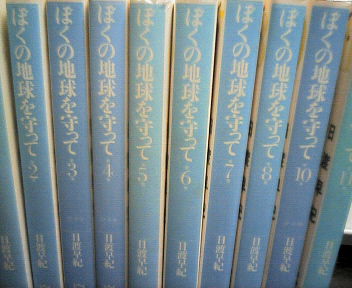This color photograph displays a row of 10 vertically standing books with their spines facing outward. The spines feature Japanese characters in a pale yellowish color and are numbered from 2 to 11, as book 1 is not visible. The books are part of a series and display various shades of blue, with the ones on the left being slightly darker, the middle ones lighter, and returning to a darker shade towards the right. All the books are uniformly designed, suggesting they belong to a cohesive collection. At the bottom right of the image, a wood floor is partially visible, adding context to the setting of this neatly arranged collection.